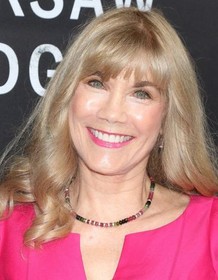This is a detailed portrait image of a Caucasian woman who appears to be around 65 or 70 years old. She has light blonde hair that is curled and falls just below her shoulders, with bangs framing her face. Her skin is fair, possibly enhanced by Botox and a facelift, and she boasts blue eyes accented by eyeliner and mascara. Her makeup includes foundation, blush, and bright pink lipstick that complements her radiant smile aimed toward the camera. She is dressed in a vibrant pink dress and wears a multicolored beaded necklace. The image captures her from a bit of space above her head to just below her collarbones. She stands in front of a black wall adorned with partially obscured white text, including discernible letters such as "K," "S," "A," "6," "O," and "G," suggesting she is at an event. Overall, she exudes a happy and glowing demeanor, indicating she is quite pleased to be at this event.